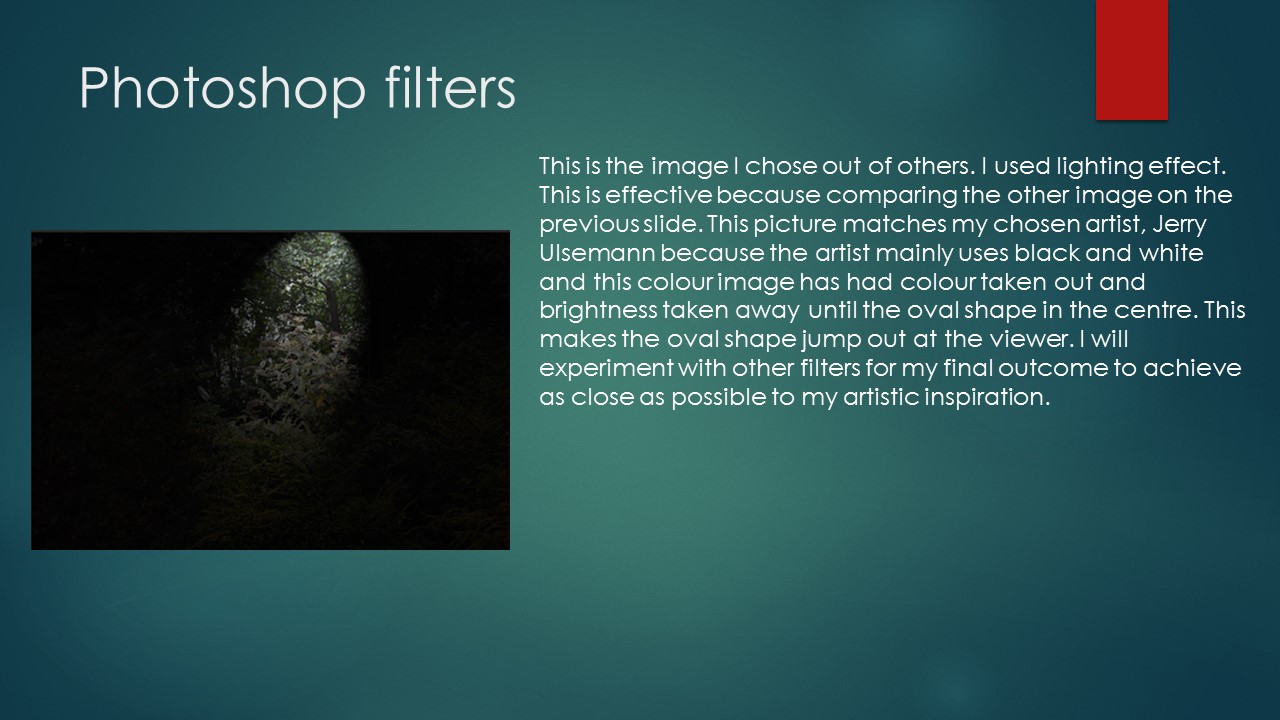This graphic is a landscape-oriented slide that resembles a PowerPoint presentation. It features a bluish background that gradients to a bluish-yellow at the center. A red vertical rectangle is placed in the upper right corner as a decorative element. In the upper left, the heading "Photoshop Filters" is displayed in white text. Below the heading, there is a black background showcasing an image that appears to be either a brown stone or light shining into a cave. To the right of the image, white text explains the image selection: "This is the image I chose out of others. I used lighting effect. This is effective because comparing the other image on the previous slide, this picture matches my chosen artist, Jerry Olsman, because the artist mainly uses black and white. This color image has had color taken out and brightness taken away until the oval shape in the center. This makes the oval shape jump out at the viewer. I will experiment with other filters for my final outcome to achieve as close as possible to my artistic inspiration."